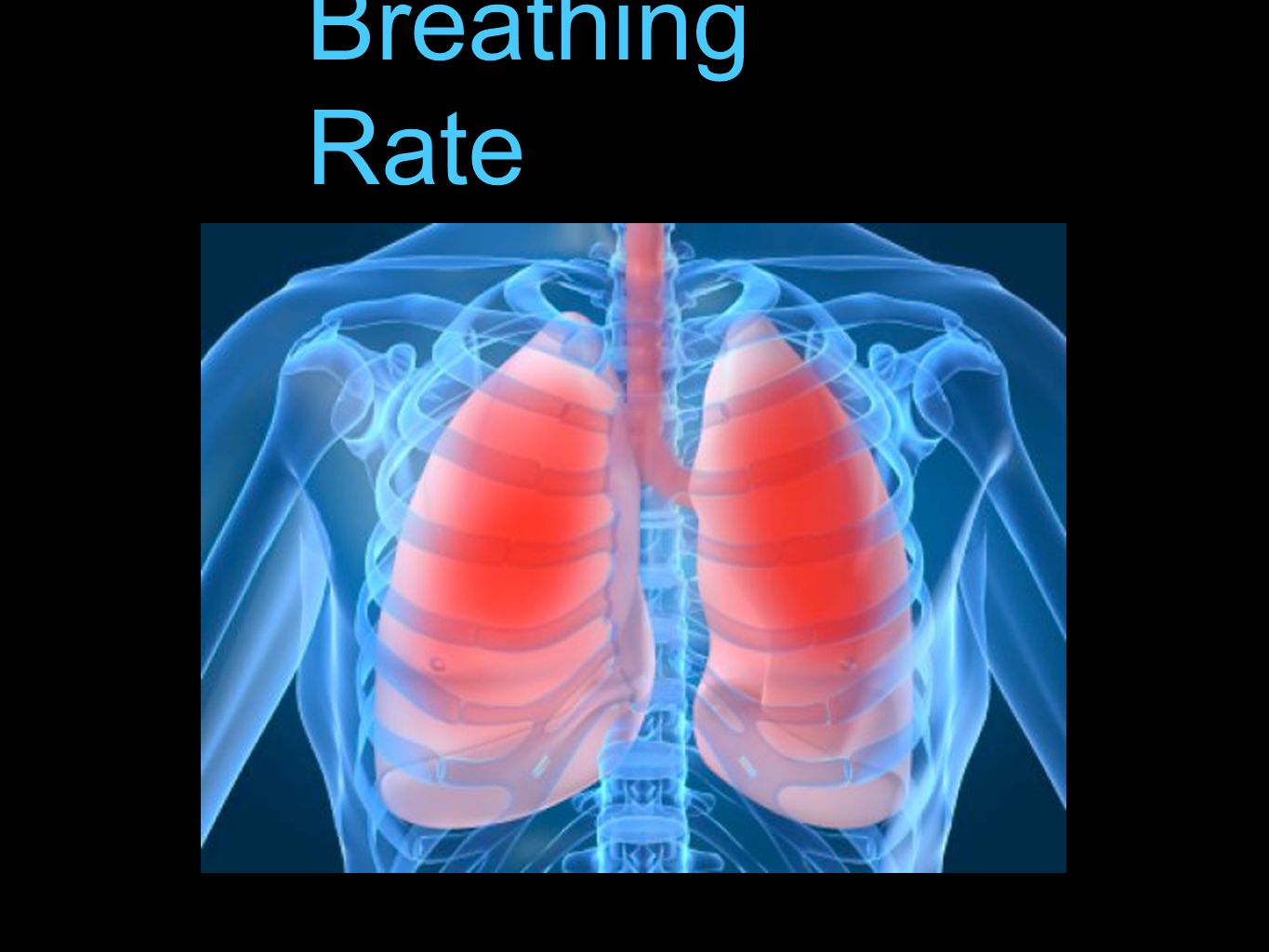This medical educational slide features a black background within a wide vertical rectangular frame, slightly wider at the top. In teal blue text at the top center of the image, though slightly left-aligned, it reads "Breathing Rate" (capital B, capital R). Below this, a smaller vertical rectangle showcases a computer-generated, digital depiction of the inside of a person's chest. The image resembles an x-ray and highlights the skeletal and respiratory systems with detailed clarity.

The bones of the ribs, shoulders, humerus, and spinal cord are illustrated in light blue. The pinkish-red lungs are prominently displayed on either side of the spinal cord, emphasizing the bronchial tubes. These tubes converge at the center and extend upwards to the trachea, suggesting the pathway to the mouth and nose. The background and general color scheme include shades of black, light blue, pink, red, and dark blue. The slide serves as a comprehensive medical visual aid, likely intended for educational purposes, such as a PowerPoint presentation.